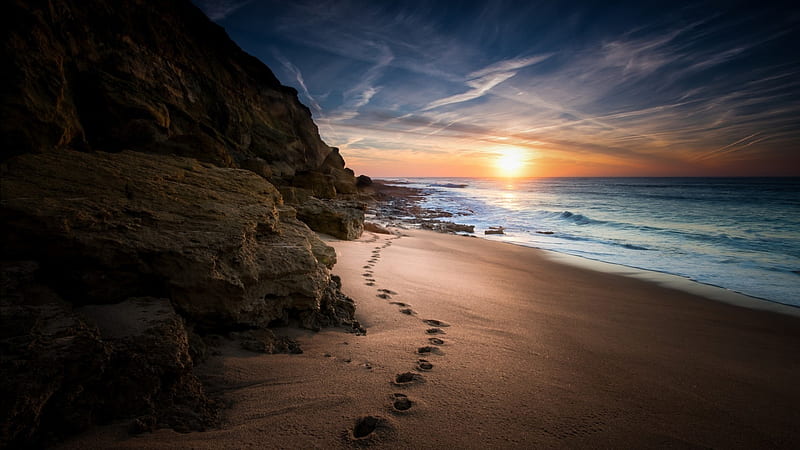A stunning painting captures the serene beauty of a sunset on a beach. The golden amber sun sinks towards the horizon, casting a warm glow across the scene. The sky transitions from a deep steel blue at the top to vibrant shades of orange and yellow nearer to the horizon, adorned with wispy white clouds that meander through the canvas. The calm, aqua-colored ocean laps gently at the shore, with small waves that hint at the incoming tide, gradually darkening to a deeper aqua green as it stretches toward the horizon.

To the left, silhouetted against the fading light, are dark, imposing rocky cliffs. In the foreground, the beach's brown sand is marked by a trail of footprints that lead towards the water and then disappear into the distance, suggesting a quiet solitary walk. Further along the beach, another set of footprints wander away, adding a sense of motion and human presence to the otherwise tranquil scene. The entire composition evokes a sense of calm and introspection, beautifully highlighting the contrasts and harmony of nature at dusk.